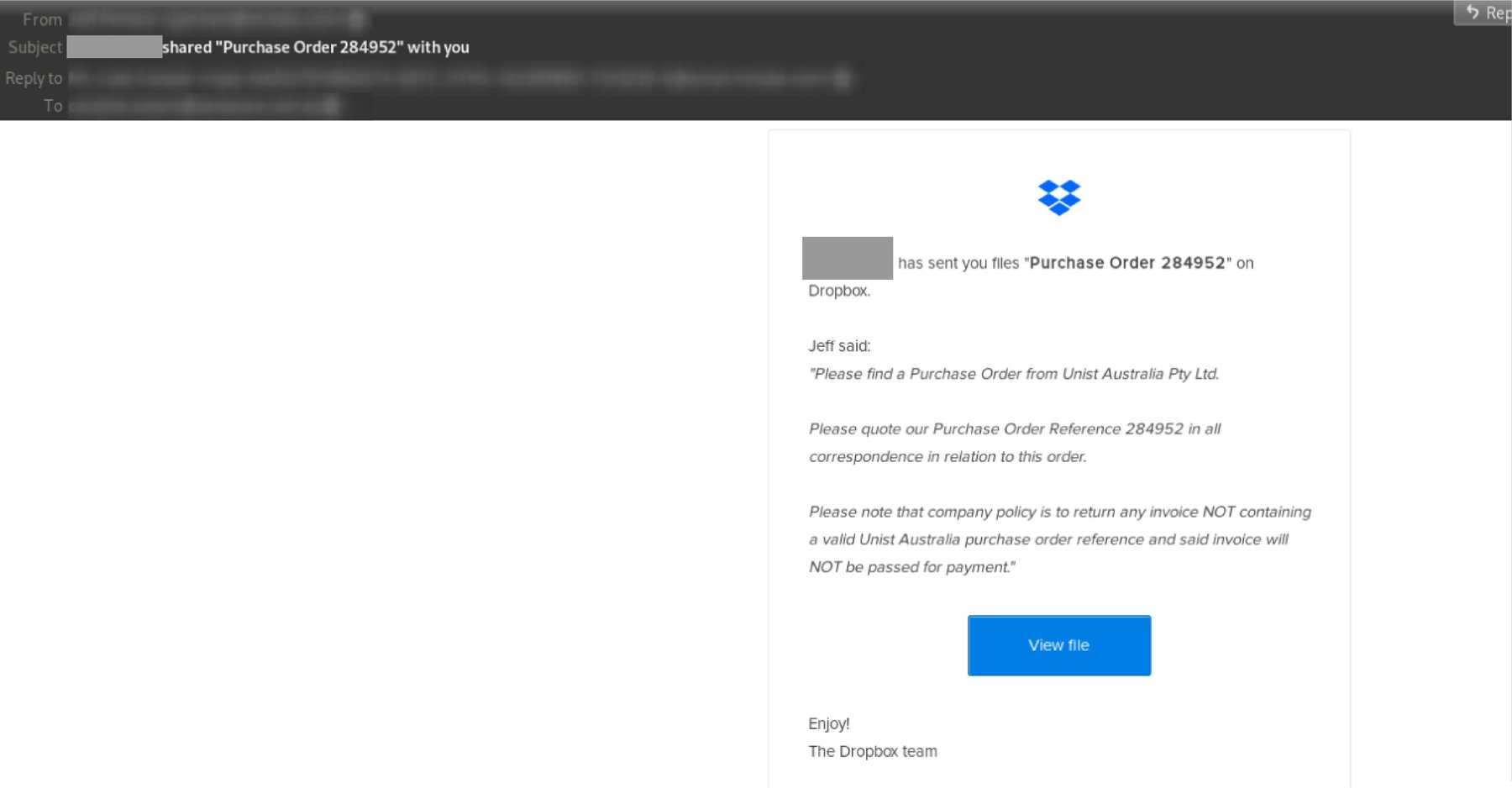In this image captured from a Dropbox email, the following details are meticulously discernible:

- **Sender and Subject Details**: The email, originating from Dropbox, appears at the top left corner. The subject line reads, "Shut Purchase Order 284952."

- **Email Content**: The central part of the email highlights the key message, which is bracketed by Dropbox's logo—a blue, open box icon to the right side. The text indicates that a file, "purchase order 284952," has been sent to the recipient. The sender, identified as Jeff, provides additional context within the email body. He states: "Please find a purchase order from Unist Australia Pty Ltd. Please quote our purchase order reference 284952 in all correspondence related to this order. Please note that it is company policy to return any invoice not containing a valid Unist Australia purchase order reference, and such invoices will not be paid."

- **Call-to-Action**: A prominent blue button, labeled "View File" in white text, is present below the email content, offering a convenient link for the recipient to access the file.

- **Footer**: At the bottom, there's a brief message from Dropbox, "Enjoy, The Dropbox Team," reinforcing the origin of the email and underscoring its professional nature.

This image represents an official communication from Dropbox about a purchase order file transfer, complete with detailed instructions and necessary compliance information.